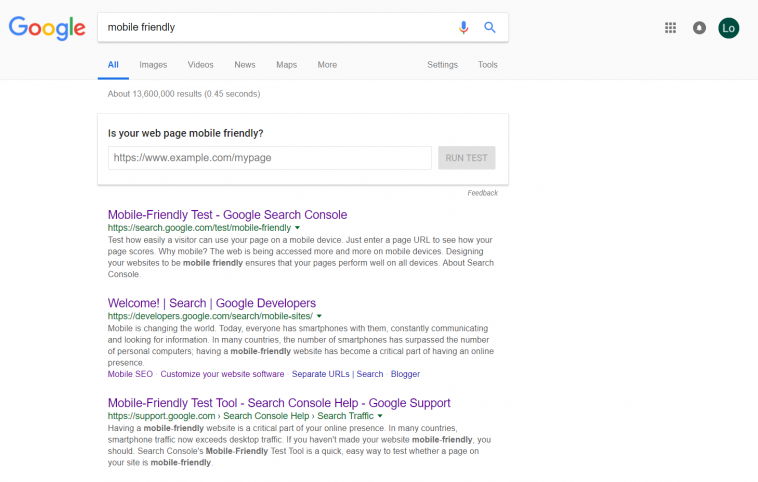The image depicts a Google search results page. In the top left corner, the recognizable Google logo is prominently displayed. The search query entered is "mobile-friendly," which is visible in the search bar. Below the search bar, several search results are listed:

1. The first result is a link for the "Mobile-Friendly Test" on Google Search Console. The description explains that this tool assesses how easily a visitor can navigate a webpage on a mobile device by simply entering the page URL.
2. The second result, titled "Why Mobile?", discusses the increasing prevalence of mobile device usage to access the web. It emphasizes the importance of designing a mobile-friendly website to ensure optimal performance across all devices.
3. The third result introduces users to the 'Search Console' and elaborates on its various functionalities.
4. The fourth result welcomes users to "Google Developers." It contains information about the transformative impact of mobile technology, noting that smartphones are now ubiquitous. The text highlights that in many regions, the number of smartphones has exceeded the number of personal computers, underscoring the necessity of having a mobile-friendly website for maintaining a strong online presence.

Overall, the search results page underscores the importance of mobile-friendly web design and provides resources for testing and improving mobile usability.